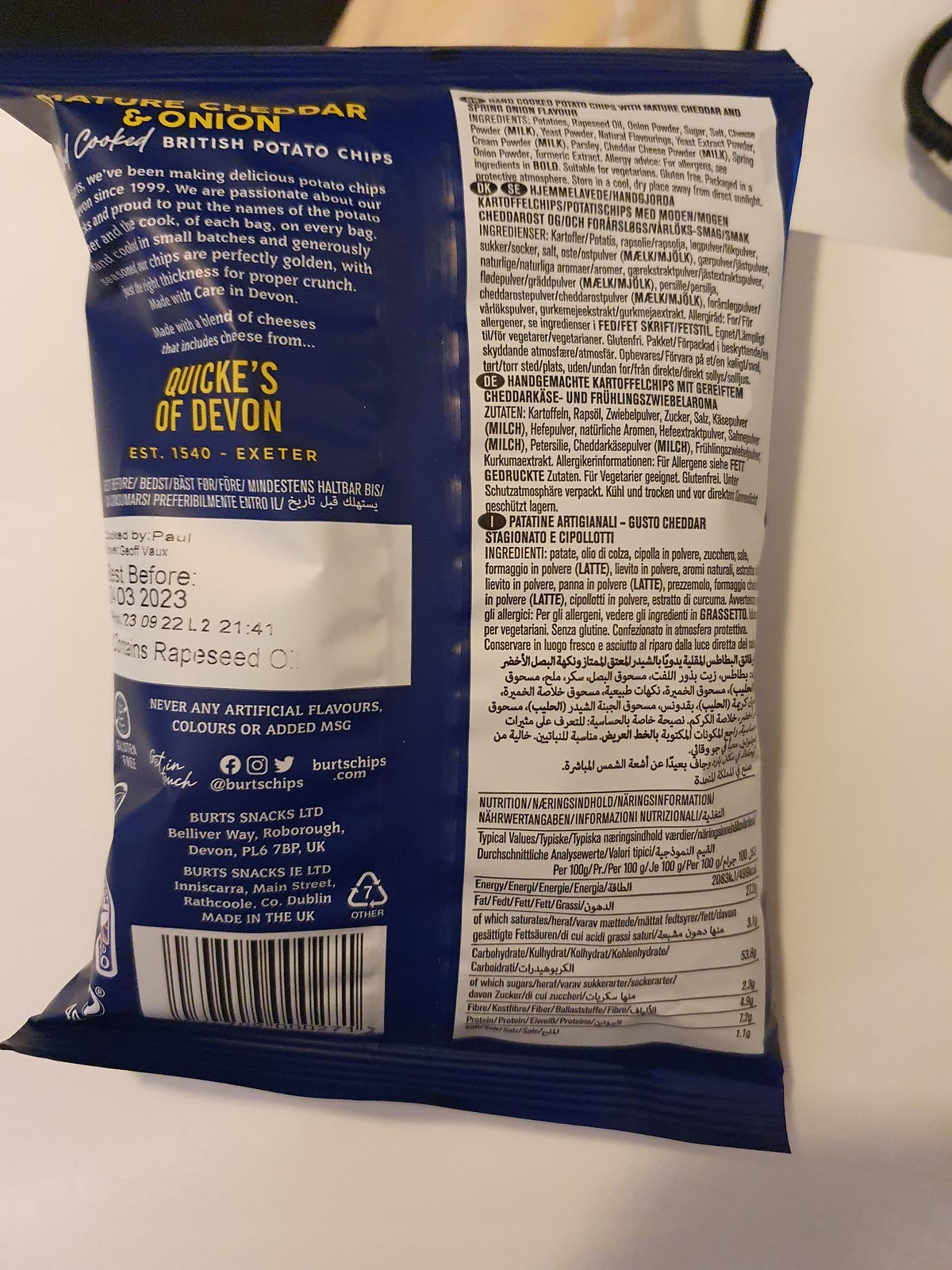This is a detailed photograph showcasing the back of a bag of British potato chips, prominently positioned on a white table or counter. The image, which is about 50% taller than it is wide, features an off-white background. The package itself is mainly dark blue. At the top left of the packaging, in large yellow text, it reads "Cheddar and Onion Cooked British Potato Chips." Below that, there's a paragraph of descriptive text. Midway down the bag in yellow letters, it says "Quickies of Devon, EST. 1540, Exeter." Adjacent to this, a white rectangular box displays a "Best Use Before" date of 03-2023. To the right side of the bag, you can see the nutrition facts and ingredients listed, which are written in multiple languages. There is also a barcode near the bottom. The background further shows the edge of the table, a tan floor, and some black elements.